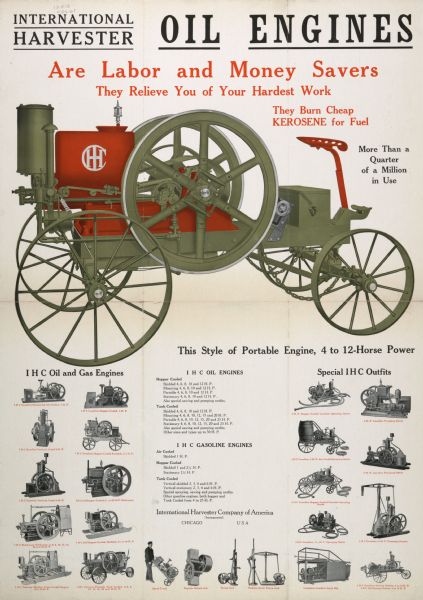The image appears to be a vintage advertisement, likely from a magazine or as a standalone flyer, showcasing diverse models of early tractors and engines. Dominated by the title "International Harvester" in prominent black letters at the top, it emphatically promotes their "Oil Engines" as both labor and money savers, claiming these machines relieve users of their toughest tasks and efficiently run on inexpensive kerosene fuel. The main focus is a large tractor with distinctive open wheels, visible pulleys, a central coil spool, an engine at the rear, and a singular metal seat at the front. The tractor is highlighted as one among 23 different models shown in smaller images below, each accompanied by text detailing specifications like the horsepower range (from 4 to 12) and the utility of the equipment. The advertisement also notes that over a quarter of a million of these machines are in use, reinforcing their widespread adoption and reliability.